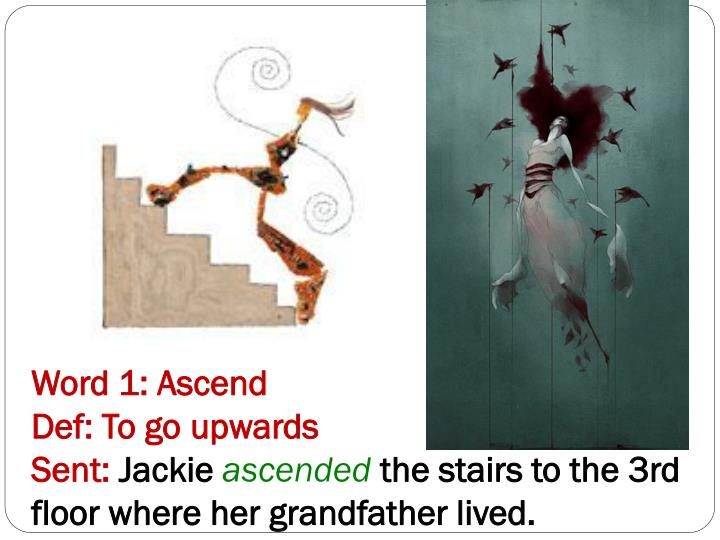The image depicts two distinct artworks accompanied by explanatory text at the bottom. 

On the left, there is a horizontally-oriented rectangular artwork showing a cartoon-like or drawing-style illustration of a figure ascending a set of stairs. The stairs are light brown, and the figure, resembling a woman, has elongated limbs with swirly, thin arms. She appears to be wearing an orange outfit with some black accents and has an orange head and long, light brown hair flowing behind her. One foot is on the base of the stairs, while the other is stretched upwards to the fourth or fifth step, emphasizing her extended, dynamic pose. Above this illustration, the text "Word: Ascend" is written in red, followed by the definition "to go upwards" and a sentence in black and green that reads, "Jackie ascended the stairs to the third floor where her grandmother lived."

On the right, the artwork showcases a more refined and different design of a woman ascending into the air. She wears a gray dress with black accents around the waistline and has voluminous, dark brown or black hair resembling cotton candy. Her elongated and ghostly figure, including disproportionately large hands and thin arms, is being lifted by at least six small black birds. The background transitions from a light mint green at the top to a darker green at the bottom, enhancing the ethereal quality of the scene.

Overall, the text below reads "Word: Ascend, Definition: to go upwards," spotlighting the theme of ascending prominently portrayed in both artistic representations.